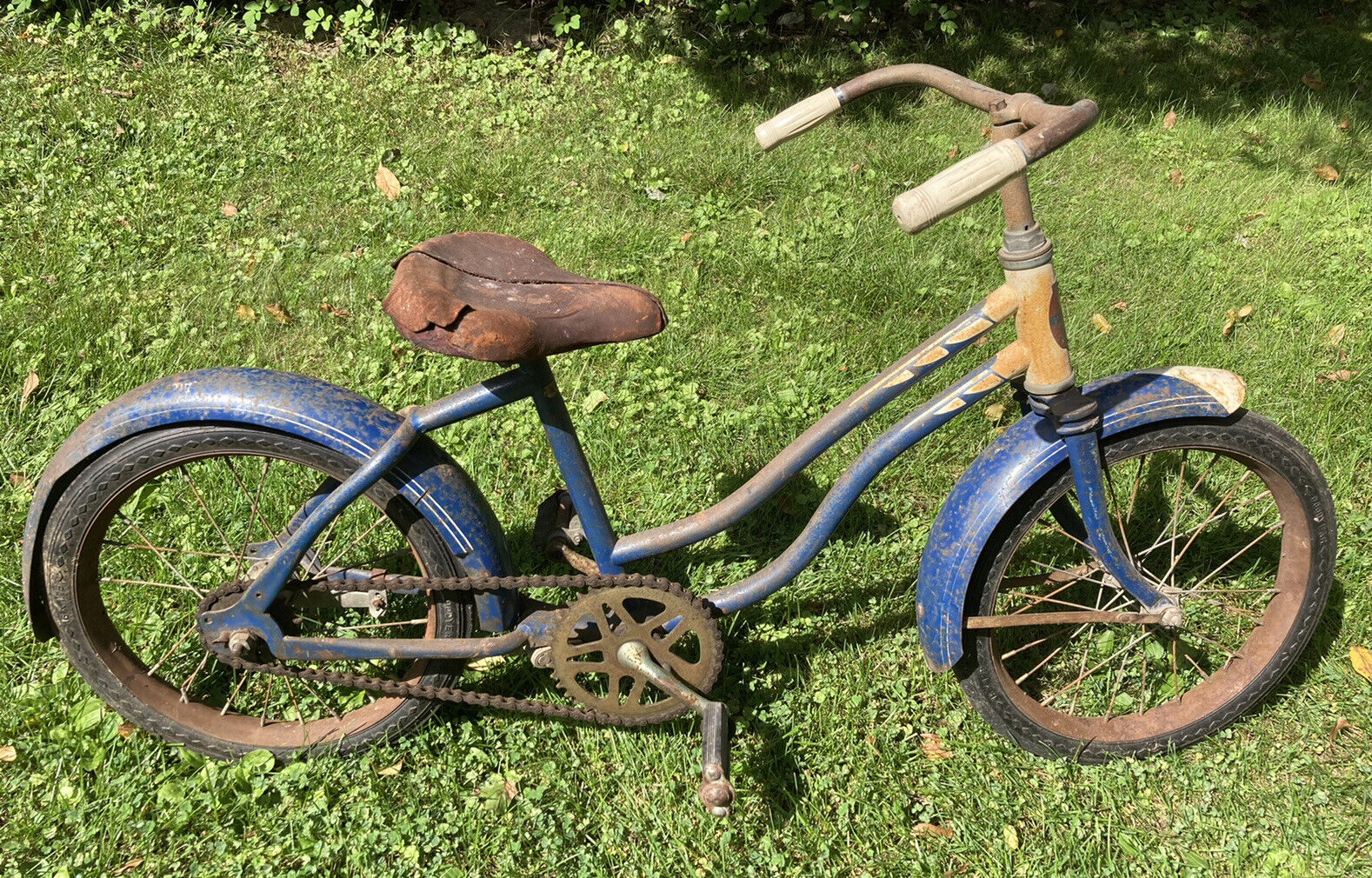This photograph showcases an antique, vintage bicycle that has clearly endured the ravages of time and exposure. The bicycle, which is predominantly blue with yellow accents near the handlebars, appears to have rusted extensively. The entire frame, chains, kickstand, and especially the seat, now cracked and separated, are all heavily corroded. The handlebars, bent into a characteristic U shape, still sport remnants of rubber grips but are enveloped in rust. The bike's tires, complete with mudguards, are similarly deteriorated, with no shine left on any part of the metal due to the extensive patina. The bicycle is positioned on a bed of green lawn, dotted with clovers, and there is a bit of shade in the top-right corner of the image, hinting at nearby trees. The overall impression is of an object left to weather the elements for many decades, with hints of its original blue and orange hues still faintly visible amidst the rust.